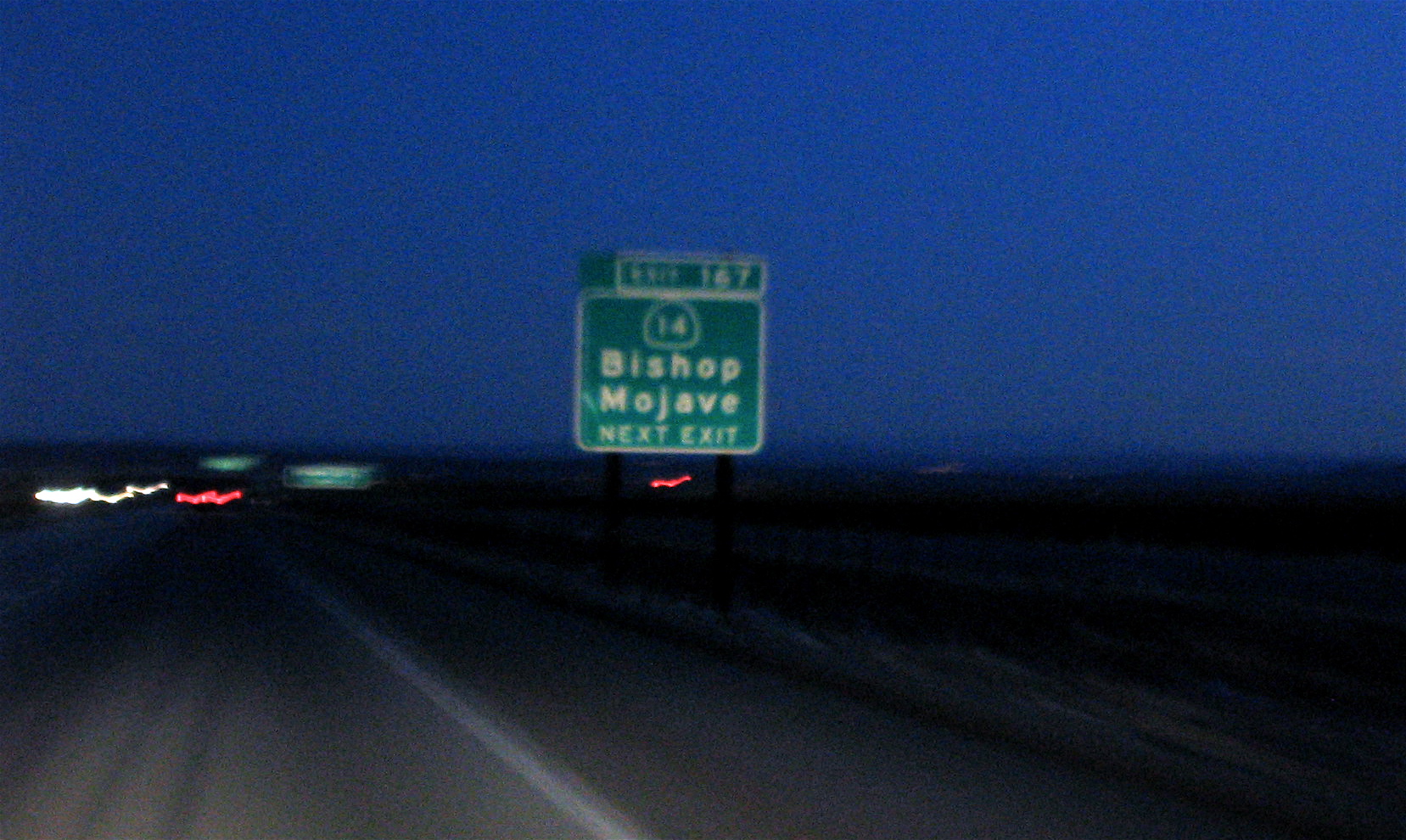A nighttime photograph depicts a blurry highway scene. On the left, the gray asphalt is marked by a diagonal white line extending from the bottom left to the center left of the image. Ahead in the distance, a horizontal stream of blurred red tail lights stretches across the highway, indicating moving traffic. To the left of these red lights, the oncoming traffic's white headlights also appear as a blurred horizontal line. Above the red tail lights, a faint green hue resembling an overhead road sign is visible. Additionally, to the right of the red lights, another green road sign appears, but both signs are extremely blurred. Dominating the center of the image is a large, heavily blurred green sign displaying white text, barely legible as "Exit 167, Route 14, Bishop Mojave Next Right." On the right side, the dark silhouette of a desert landscape merges with the rich, deep blue sky above, adding to the overall mystique of the scene.